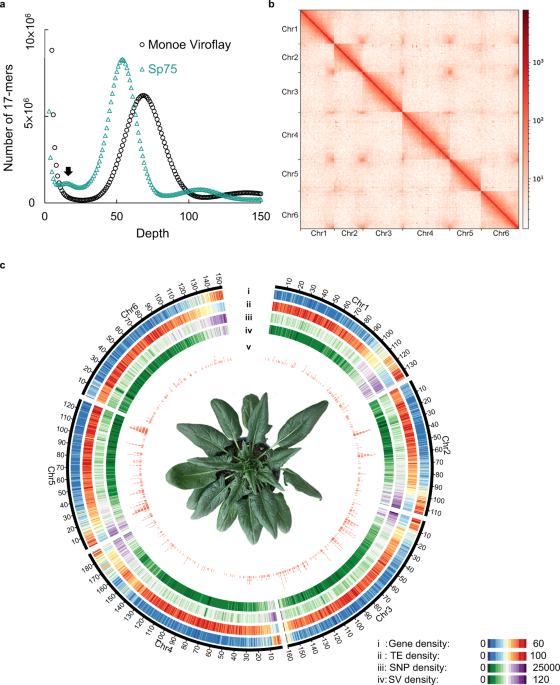The image showcases three distinct graphical presentations. The top left graphic, labeled "Monroe Veroflay," features a detailed chart with a 90-degree plot displaying the "number of 17 mers" on the y-axis, ranging from 0 to \(10^6\), and "depth" on the x-axis, from 0 to 150. The data is illustrated with green and black controls. Adjacent to it on the top right, another graph with a tan background and shades of pinks and oranges, marked as "CHR123456," echoes the format but includes a prominent red line running diagonally from the top left to the bottom right corner, suggesting a different set of data parameters. The bottom graphic is a vibrant, multi-colored circular chart centered around a plant in a blue pot. This circular chart is segmented with varying degrees of greens, purples, blues, oranges, and reds, each ring indicating densities such as gene density, TE density, SNP density, and SV density. The intricate design and color gradients provide a comprehensive visual representation of the data.